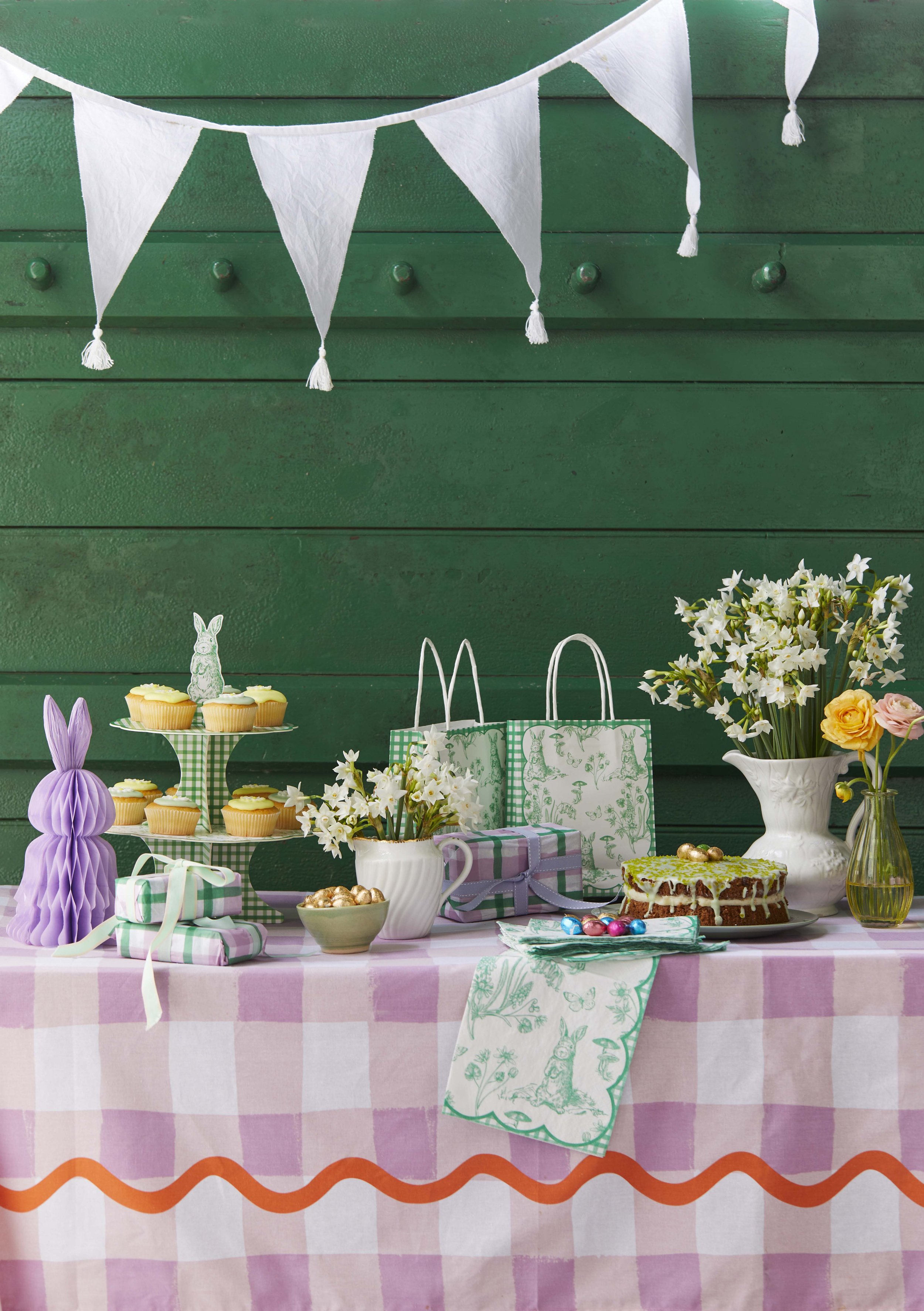This indoor color photograph showcases an elaborately decorated Easter-themed banquet setup. The long table at the bottom of the image is draped with a purple and white checkered tablecloth, featuring an orange zigzag trim at the base. Arranged atop the table is a festive assortment of Easter decorations and goodies. Central to the display is a two-tiered cupcake stand with a green and white checkered frame, adorned with lightly frosted white cupcakes crowned with an Easter bunny figure. Flanking the cupcakes are various presents in plaid wrapping and gift bags, with two presents notably stacked.

A centerpiece of the table is an Easter cake, artfully unfrosted on the sides with a drip effect and topped with decorative mini gold eggs. Scattered around are wrapped Easter egg candies in cheerful pastel wrapping. In terms of floral decorations, the table features a vase with light daisies and a clear vase with a couple of tulips, adding a fresh spring touch.

The backdrop highlights a green wall embellished with a party streamer and a white flag banner strung across the top, enhancing the celebratory atmosphere. This setup, adorned with details such as a paper lavender rabbit and decorative napkins, embodies the joyful spirit of an Easter gathering.